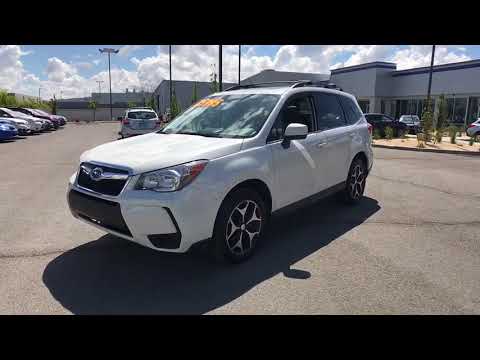In this detailed image, we see a white Subaru Forester, possibly from 2014 or 2015, parked in the middle of a lot, likely a car dealership parking area. The vehicle, captured from a front driver's side angle, features a yellow, possibly price-related, sticker on the top left of its windshield. The large black wheels with silver spokes and some black accents on the front part of the car are evident. The bright, sunny day casts sharp shadows beneath the car, highlighting the clear blue skies and big, white clouds. In the background, there is a substantial white-painted, one-story building and scattered light poles typical of a dealership and maintenance facility. Farther back, several cars are noticeable, including a red and a blue car, along with additional white vehicles. The entire scene is framed by a black border, emphasizing the well-maintained environment and the short plants visible in the distance.